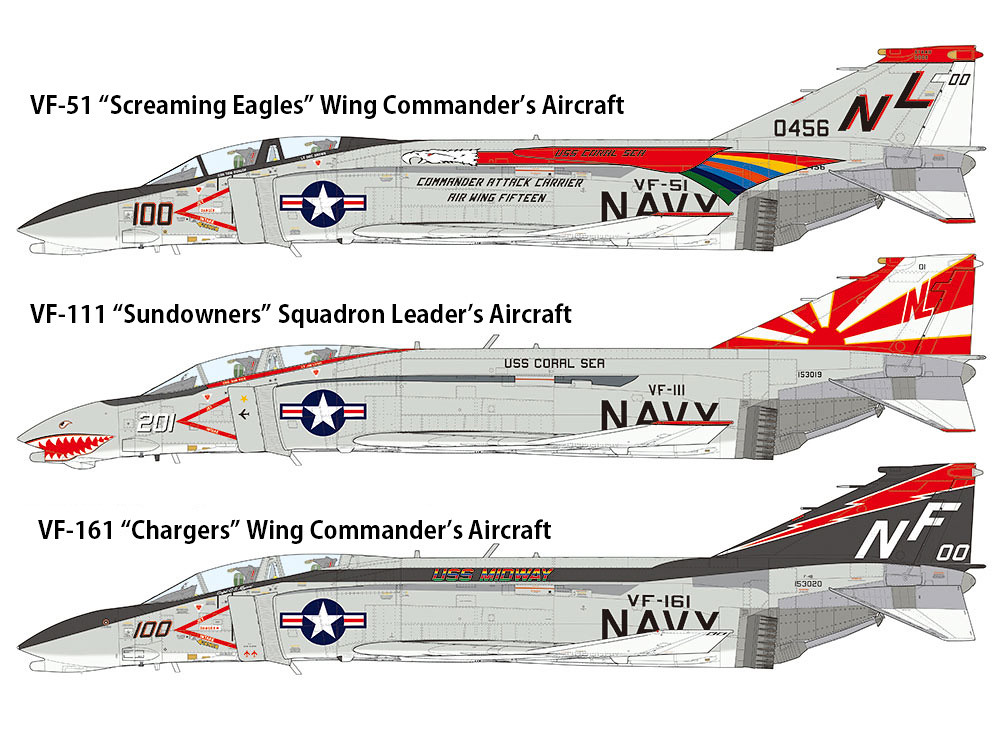The image is an illustration featuring three military aircraft, all depicted in gray with distinctive designs and markings. 

The first aircraft is the VF-51 Screaming Eagles Wing Commander's aircraft. It features a detailed white-headed eagle with a red body, and a colorful tail in red, yellow, blue, orange, navy blue, and green. The body of the aircraft bears the labels "Commander, Attack Carrier Air Wing 15", "VF-51 Navy", "USS Coral Sea", and "D-456NL". It also sports the aircraft number "100" near the front, a white star in a blue circle flanked by red, white, and blue stripes, and rainbow stripes near the tail.

The second aircraft is the VF-111 Sundowners Squadron Leader's Aircraft, which features a simpler design but includes a striking shark face on the front. Labeled with "201", it prominently displays the red, white, and blue star logo, "USS Coral Sea", "BF-111 Navy", and "153019" near the tail. The tail itself showcases a red dot with emanating red and white beams and the letters "NL".

The third aircraft, VF-161 Chargers Wing Commander's Aircraft, also features a simpler design with the aircraft number "100" on the front and the red, white, and blue circle logo. It includes the labels "USS Midway" in rainbow colors, "BF-161 Navy", "153021" near the tail, "NF-00" on the tail, and a red and white lightning bolt. 

The illustration is a colorful and detailed representation of these three distinct naval aircraft, each with unique markings denoting their respective squadrons and commands.